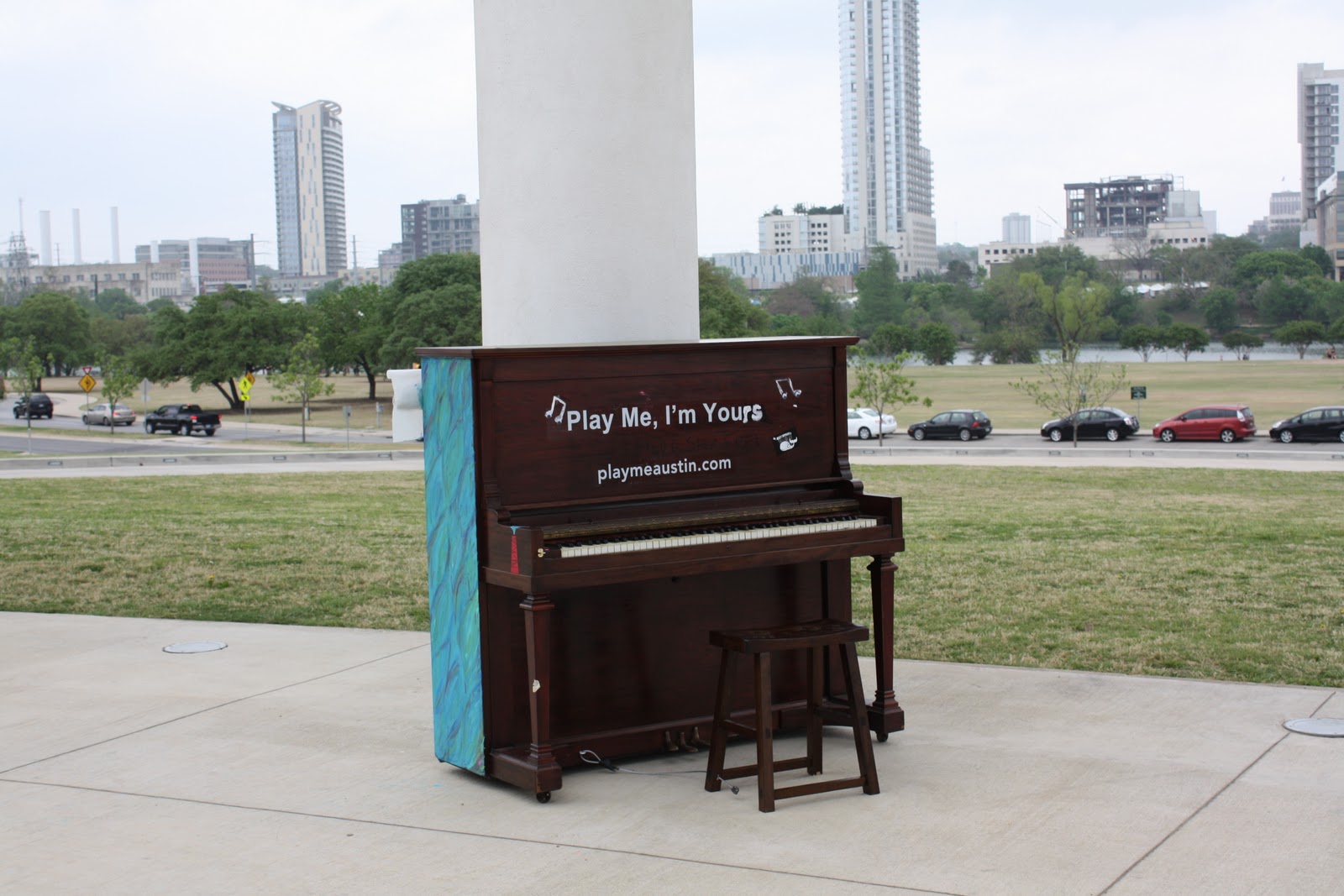The photograph captures an outdoor piano placed prominently on a gray concrete surface, positioned in front of a large, white-painted cylindrical concrete support beam. The piano, crafted from dark brown wood, has a rectangular shape and features a small, backless brown wooden bench situated in front of it. The keys are a contrasting combination of white and black. The words "Play Me, I'm Yours" are inscribed in white text on the upper part of the piano, flanked by white music notes, with the website "playmeaustin.com" written beneath the phrase. Blue cloth drapes on the sides of the piano, adding a splash of color. Surrounding the piano is a broad concrete area backed by a patch of green grass, and beyond that, a cityscape unfolds with a street bustling with cars and a skyline dotted with high-rise buildings and skyscrapers, including a parking garage. The scene seamlessly blends urban life with the inviting charm of the musical instrument.